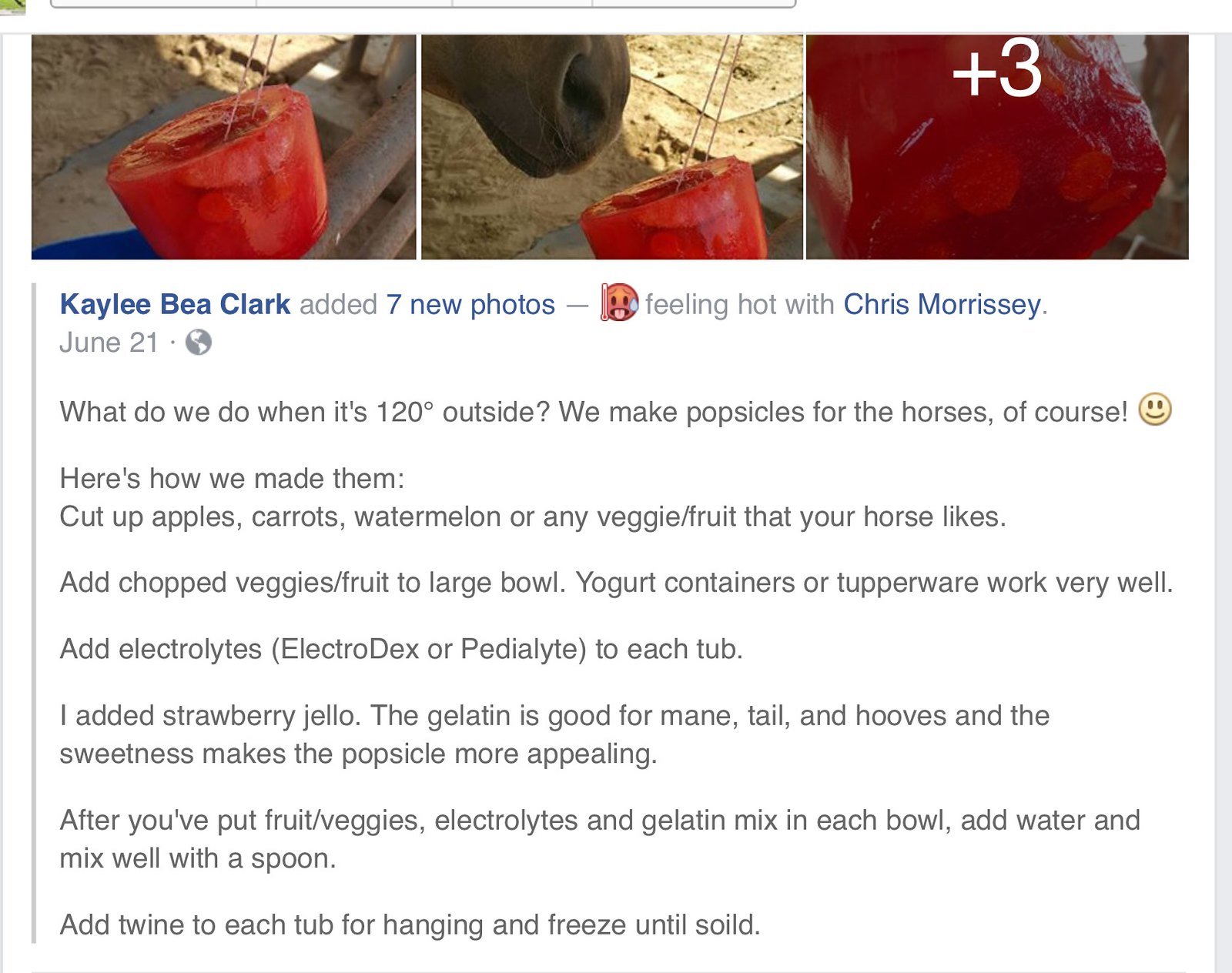In a Facebook post from June 21st, Kaylee Bay Clark, feeling the heat with Chris Morrissey, describes making popsicles for their horses to combat the 120-degree weather. The post contains three photographs: the first shows a little red bucket, the second captures a horse approaching the bucket, and the third provides a close-up of the bucket. The detailed caption explains the process: cut up apples, carrots, watermelon, or any fruit and veggies your horse likes, and place them in a large bowl or yogurt containers. Add electrolytes (such as Electrodex or Petalite) and strawberry jello for its benefits to mane, tail, and hooves and for added sweetness. Mix everything with water in the containers, then attach twine for hanging and freeze until solid. The post highlights a creative and practical way to keep horses cool during extreme heat.